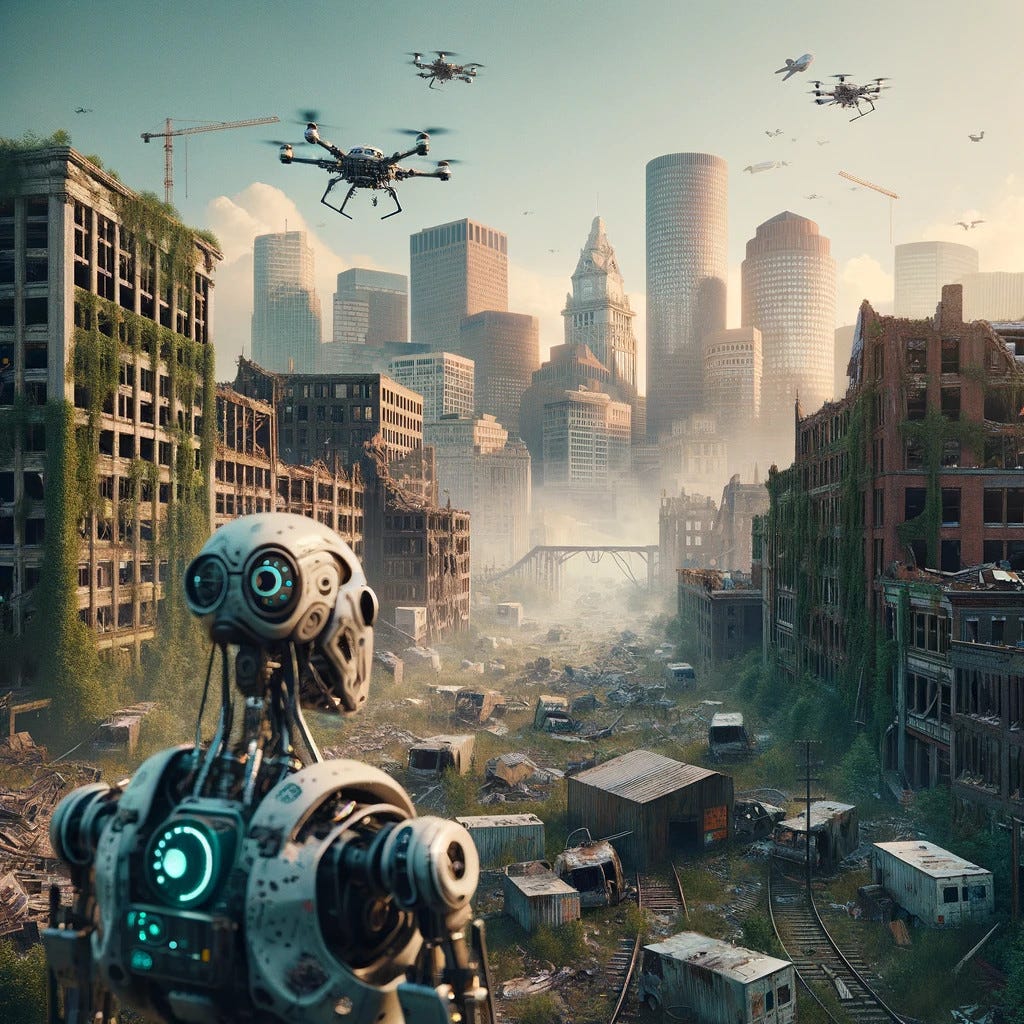The image depicts a digitally created, post-apocalyptic, futuristic world. Dominating the foreground, a skeletal, humanoid robot with mechanical gears and dials for eyes stands facing a desolate street. The street, overtaken by moss, ivy, and other greenery, is cluttered with abandoned, burnt-out vehicles and sections of railroad tracks partially buried under the overgrowth. To either side of the street, dilapidated buildings are covered in vines and moss, suggesting years of abandonment and decay. Further down the street, a damaged bridge can be seen amidst the devastation. 

The scene is punctuated by robotic helicopters, reminiscent of spiders, hovering above, with propellers on each of their extended arms. These drones seem to be the agents of destruction. In the distance, a skyline of tall, more futuristic buildings looms, partially obscured by a smoky mist rising from the debris below. Above this chaotic tableau, the sky remains eerily calm, a stark blue with light clouds. The overall scene evokes a sense of a once-bustling urban area now desolated and overtaken by both nature and advanced robotics.